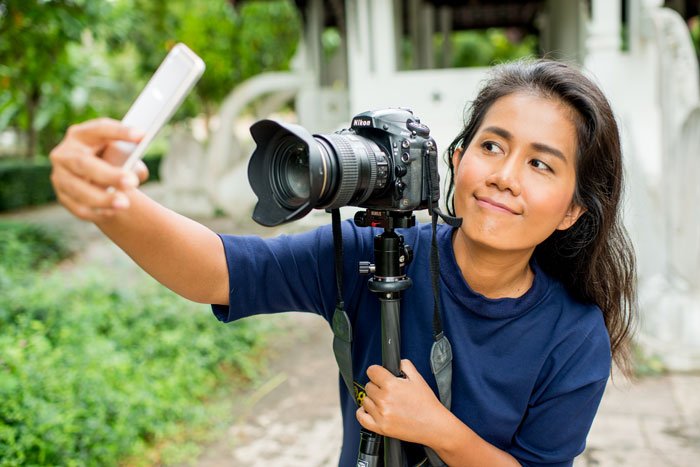In this captivating photograph, a woman in her 30s, possibly of Asian descent, stands outdoors in a garden area holding a Nikon professional camera mounted on a tripod. She has long, dark, loose hair with hints of gray and a tan complexion. Dressed in a blue short-sleeved top that reaches her elbows, she manages the camera with one hand gripping the tripod, while her right hand holds a smartphone. This intriguing setup appears as though she is using her professional camera to take a picture of herself through her smartphone, which adds a multi-layered depth to the imagery. Her expression is a mix of focused intent and subtle satisfaction, suggesting she is pleased with what she is capturing. The background showcases a blurred, white building, possibly a cottage or a small cathedral, surrounded by tall trees, a hedge, and some shrubbery. The image encapsulates a moment where modern technology meets professional artistry, creating a unique and visually compelling self-portrait in a lush, serene environment.